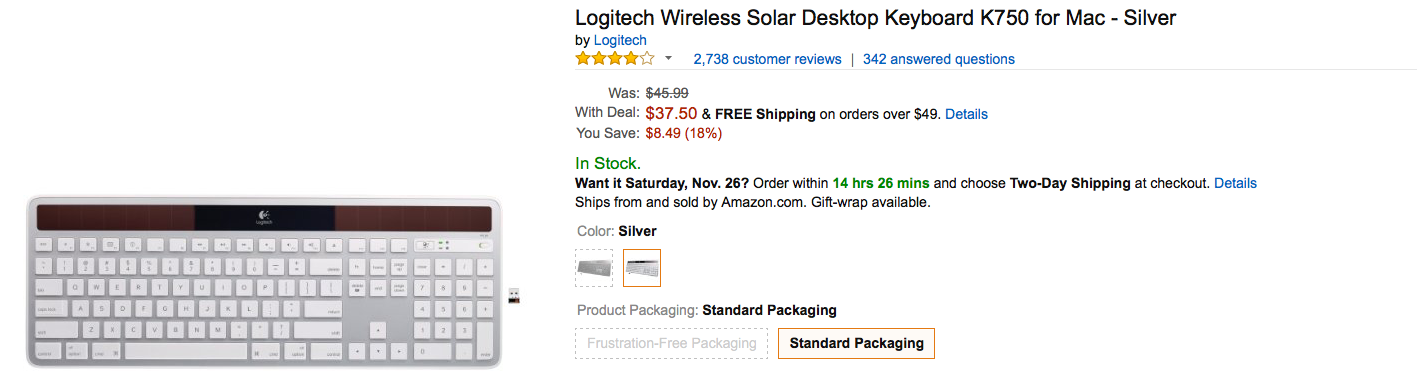### Product Description for Logitech Wireless Solar Desktop Keyboard K750 for Mac

Presented is a detailed product listing for the Logitech Wireless Solar Desktop Keyboard K750 for Mac, in silver, displayed on an Amazon page.

- **Product Title**: Logitech Wireless Solar Desktop Keyboard K750 for Mac - Silver
- **Brand**: Logitech (clickable link to the brand's page)
- **Customer Ratings**: 4-5 stars, based on 2,738 customer reviews (clickable), and 342 answered questions (clickable)
- **Pricing**: 
  - Regular Price: $45.99
  - Discounted Price: $37.50 
  - Savings: $8.49 (18%)
  - Free Shipping on orders over $49 (clickable "Details" link)
- **Availability**:
  - Status: In Stock (text in green)
  - Estimated Delivery: Saturday, November 26
  - Urgency Note: Order within 14 hours and 26 minutes and choose two-day shipping at checkout (clickable "Details" link)
  - Ships from and Sold by: Amazon.com 
  - Gift wrap availability mentioned
- **Color Options**:
  - Primary: Silver
  - Alternative Color: Another color option listed but not selectable
- **Packaging Options**:
  - Selected: Standard Packaging
  - Unavailable Option: Frustration-Free Packaging (non-selectable)
- **Product Image**: 
  - A visual on the left side showing a silver keyboard with white keys and a dark bar along the top, which is presumably a solar panel.

This detailed caption provides a comprehensive overview of the product, its purchasing options, and additional details, enhancing clarity for potential buyers.